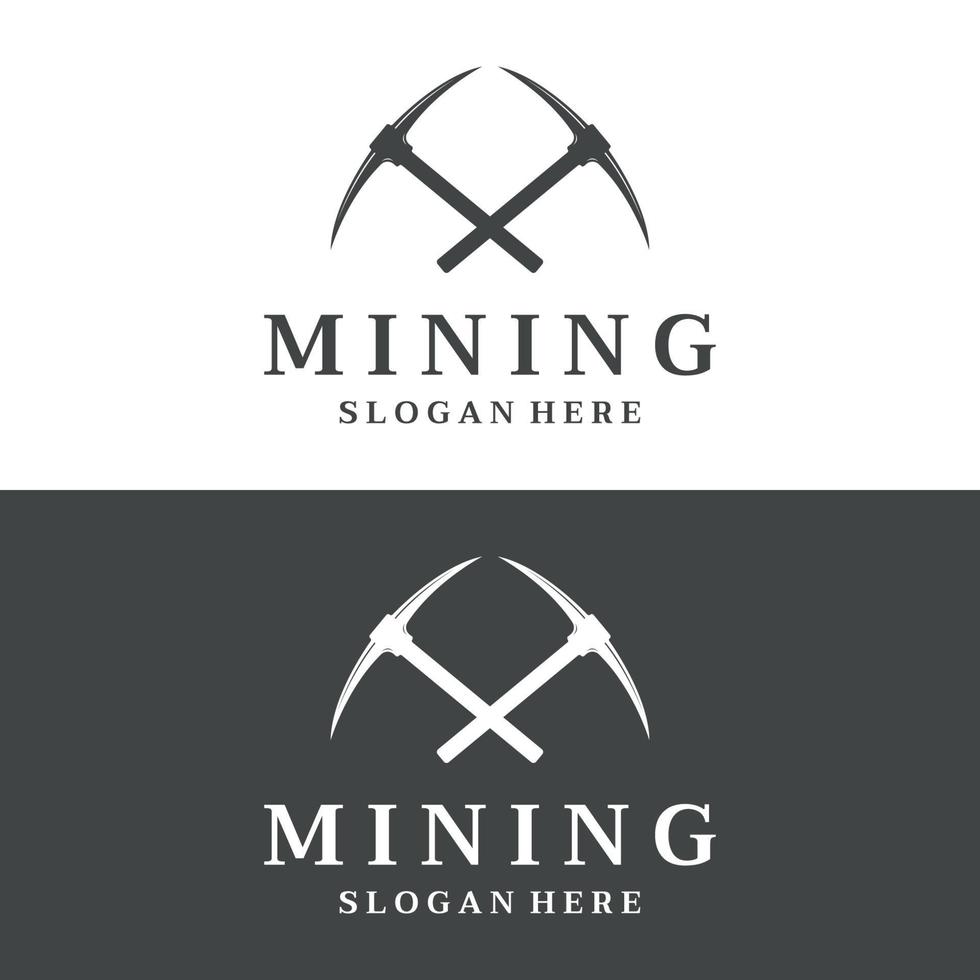The image features two distinct alternate designs, likely prototypes for a mining company's branding. The top design showcases two gray pickaxes crossing each other on a white background with the text "Mining Slogan Here" written in black below it. In contrast, the bottom design mirrors the top but with the colors inverted: it displays two white pickaxes crossing each other on a dark gray background, with the same text "Mining Slogan Here" in white. Both designs feature the same font size for the text and have no additional words or pictures. The pickaxes, detailed with wood handles and iron heads, symbolize typical mining tools, emphasizing the mining theme of the potential branding.